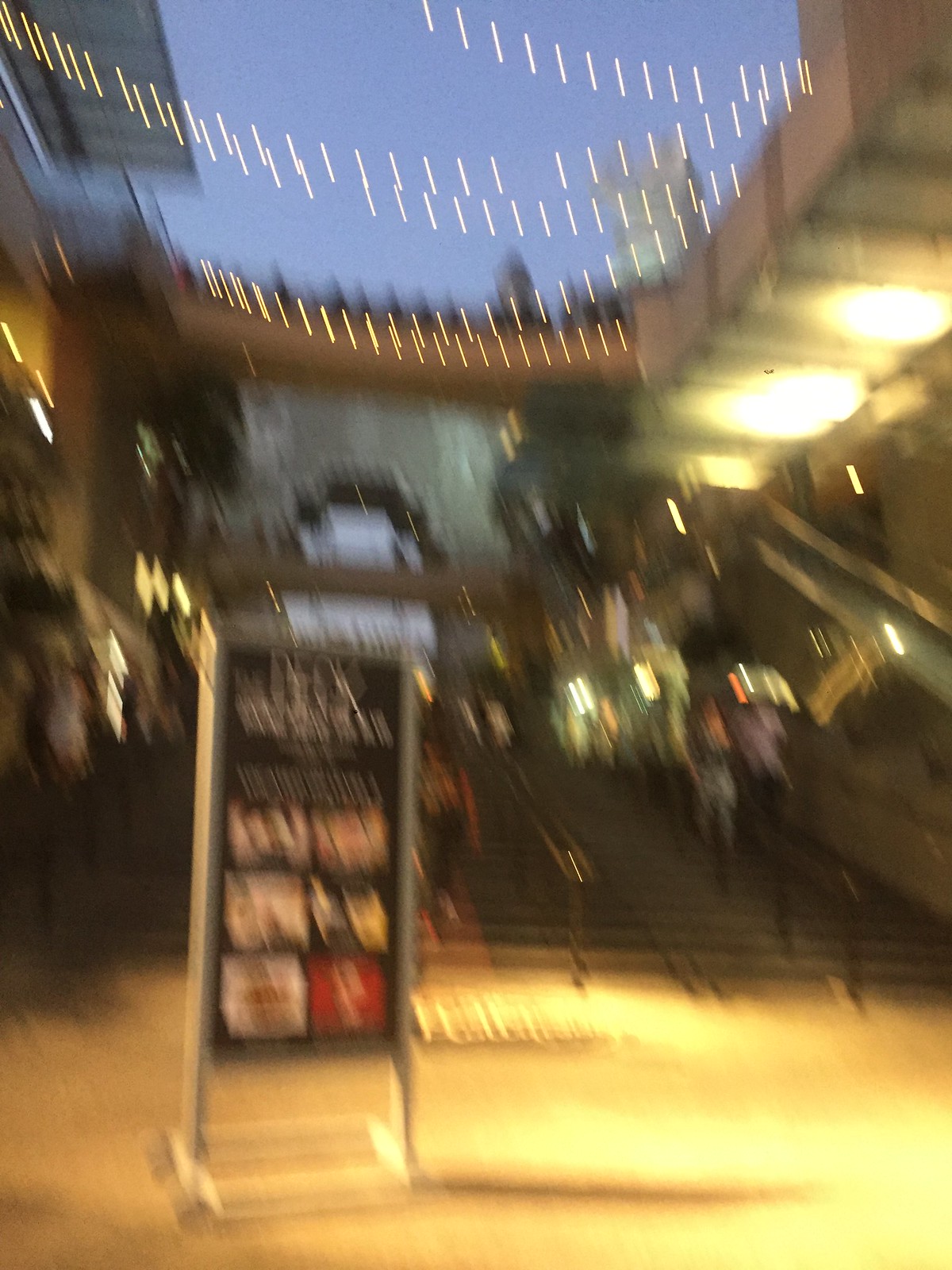In this blurry nighttime image of an old town centre, we observe a small, quaint street flanked by shops and restaurants. The scene is accentuated by a long exposure effect, giving it a dreamy, indistinct quality. Dominating the foreground, a visible restaurant menu on the left cannot be read due to the blurriness. In the middle of the image, a ramp and dark grey stairs ascend towards what appears to be an indoor area, possibly a mall or dining area. People are seen walking up and down the ramp and stairs, though their details are obscured by the blur. Overhead, large lights and fairy lights strung across add to the ambiance. An exposed ceiling reveals a glimpse of the blue night sky above. On the right side of the image, an escalator is visible, contributing to the bustling atmosphere. Near the base of the staircase, a tall rectangular sign with a grey frame and black surface features six indistinct pictures and unreadable text in white. The scene evokes a lively business courtyard or entertainment district, decorated with festive Christmas lights hanging from the rafters amidst the bustling crowd.